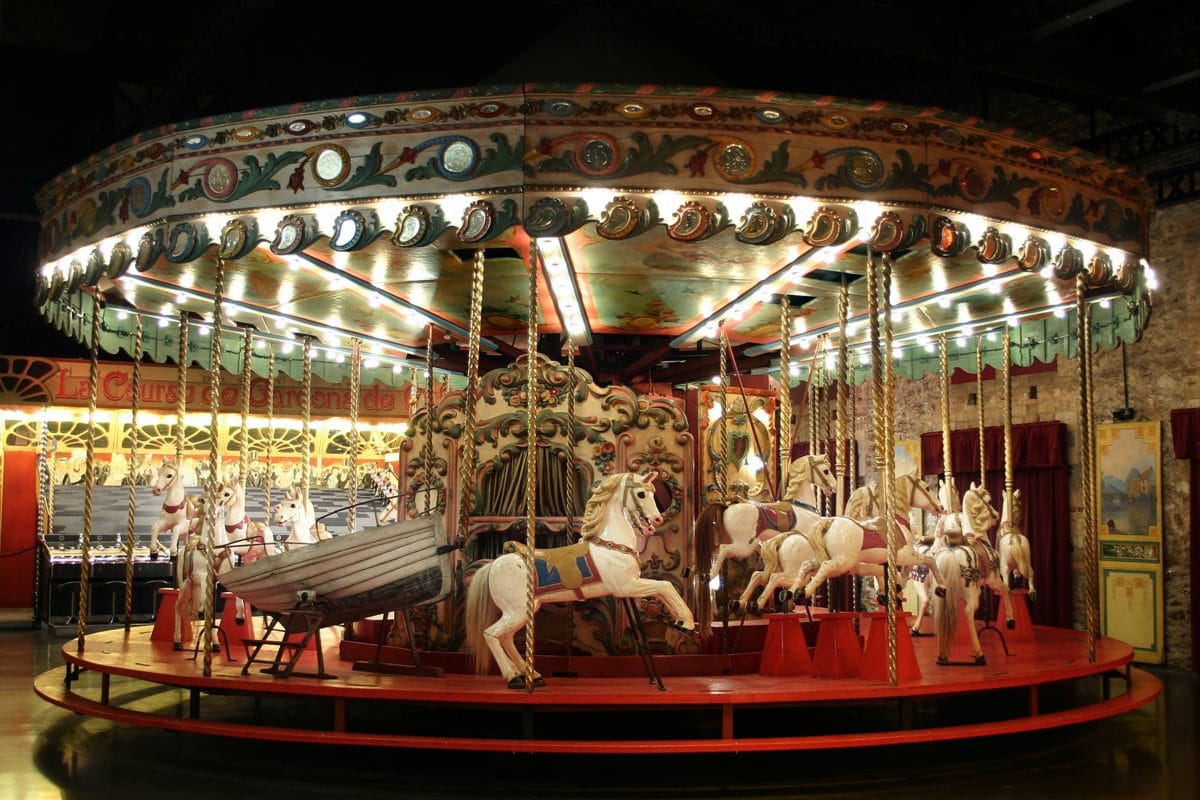This photograph captures a beautifully illuminated, old-fashioned round carousel against the backdrop of a dark night sky. The carousel, fully lit and meticulously clean, stands empty with no people in sight. It features a red wooden base and platform that wraps around its circumference. Adorned with white horses, each with blonde manes and tails, the carousel also includes a unique white boat with a little black ladder amidst the horses. Golden poles extend up and down between the horses and the boat. The top of the carousel boasts elaborate engravings in white and green, accentuated by bright white lights. The background reveals intricately designed walls with carvings of green leaves and pink flowers, contributing to the carousel's ornate and nostalgic appearance.